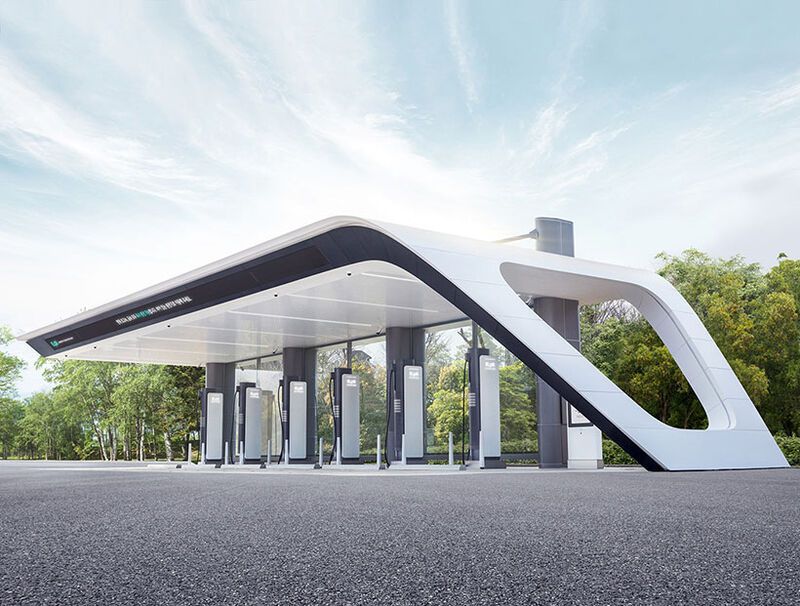In this image, we see a futuristic charging station for electric vehicles, characterized by a sleek, spaceship-like white dome structure with a label featuring text that is too blurry to read. The station comprises six or seven silver charging outlets, arranged in a line across the width of the structure. The ground beneath the station is a typical gray parking lot asphalt, accompanied by patches of gravel. The low-angle camera shot reveals a backdrop of lush trees, framing the station against a sky filled with wispy white clouds over a blue horizon. The station stands alone without any attached convenience store, highlighting its modern and functional design in a scenic outdoor setting.